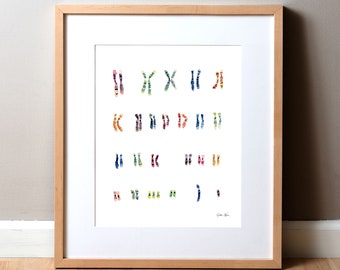This framed piece of artwork, suitable for a nursery, is a detailed and intricate visual representation of a family's DNA lineage, spanning multiple generations. The light brown wooden frame encloses a white mat, providing a contrasting border to the intricate design within. The artwork features a pattern reminiscent of an eye chart, with symbols or letters that appear to decrease in size from top to bottom. These symbols could represent DNA chains, tracing the genetic connections from ancestors down to the newest family member, emphasizing the continuity of the family line. Though the overall image quality is somewhat low and gives off a blurry appearance, the subtle details include a light grayish background with a delicate white overlay and black initials in the bottom right corner. The artwork's base sits on a light brown ground, with a light gray wall behind it, adding to the piece's serene and soft aesthetic suitable for a child's environment.